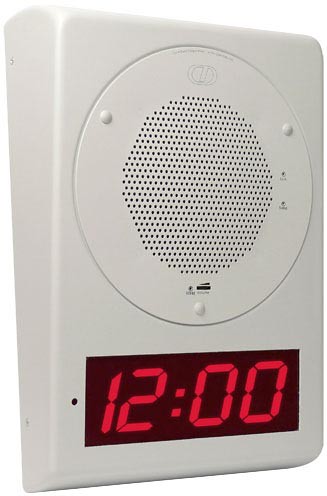This image features a white device that appears to be a combination of a wall clock and a speakerphone. The main body of the device is white, and at the bottom, there is a clock with a dark red background and red numerals displaying the time as 12:00. Above the clock face, there is a speaker section equipped with a volume meter at the bottom, allowing for the adjustment of sound levels. On the right side of the speaker, two auxiliary ports are visible. Additionally, the brand logo, characterized by a 'T' encircled, is situated at the top of the product.